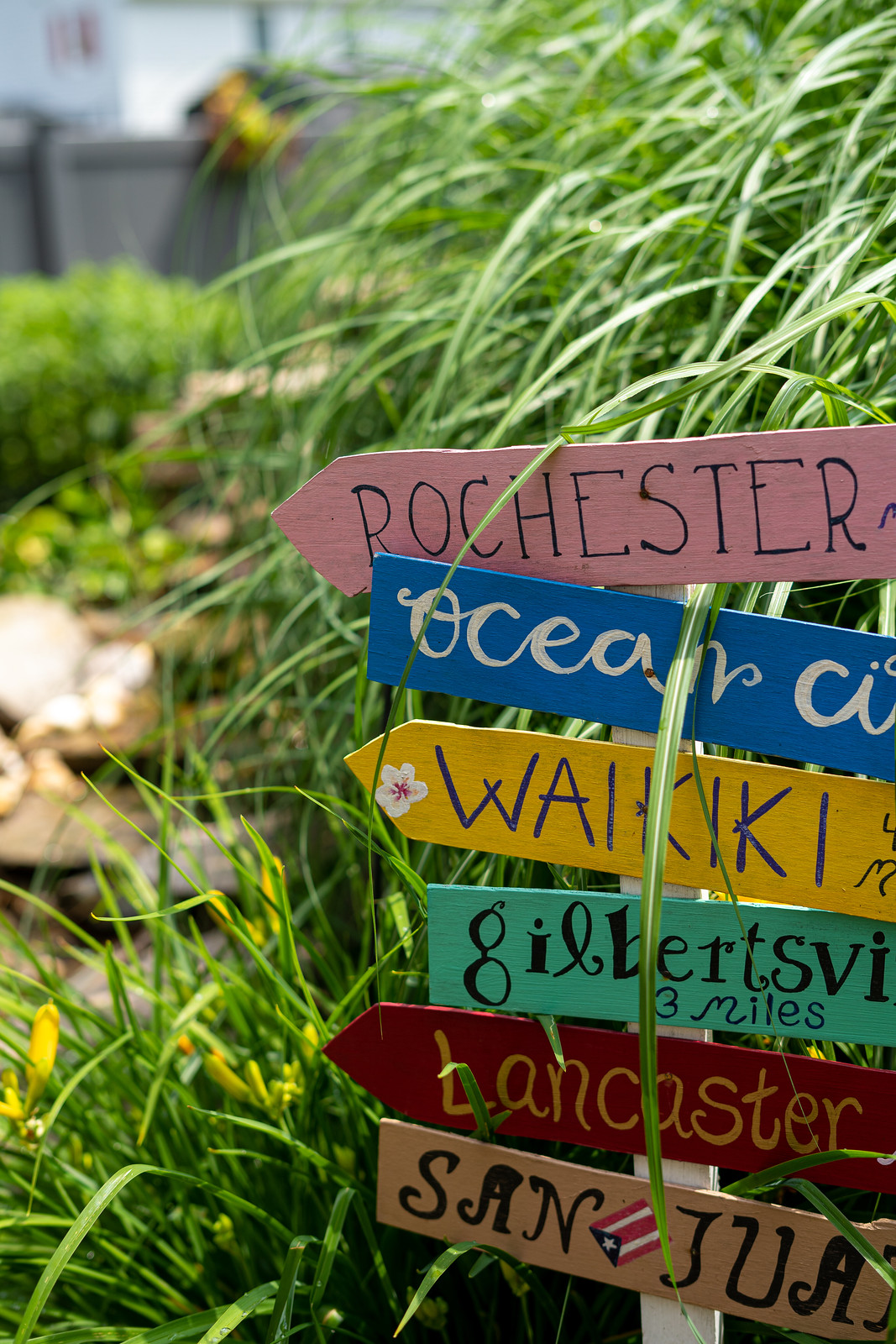In this vibrant garden scene, the focal point is an eclectic signpost resembling a traditional weather vane, composed of six different colored mini signs. Each sign, marked with a distinct city name, points in a different direction. From top to bottom, the cities are Rochester in pink, Ocean City in blue, Waikiki in yellow, Gilbertsville in green, Lancaster in red, and San Juan in brown. Notably, the San Juan sign features the Puerto Rican flag, adding a charming and homey touch. The signs are set amidst overgrown grass and various plants, spilling onto a pathway of stones. In the background, a blue fence and some steps are visible, contributing to the garden's cozy and whimsical atmosphere.